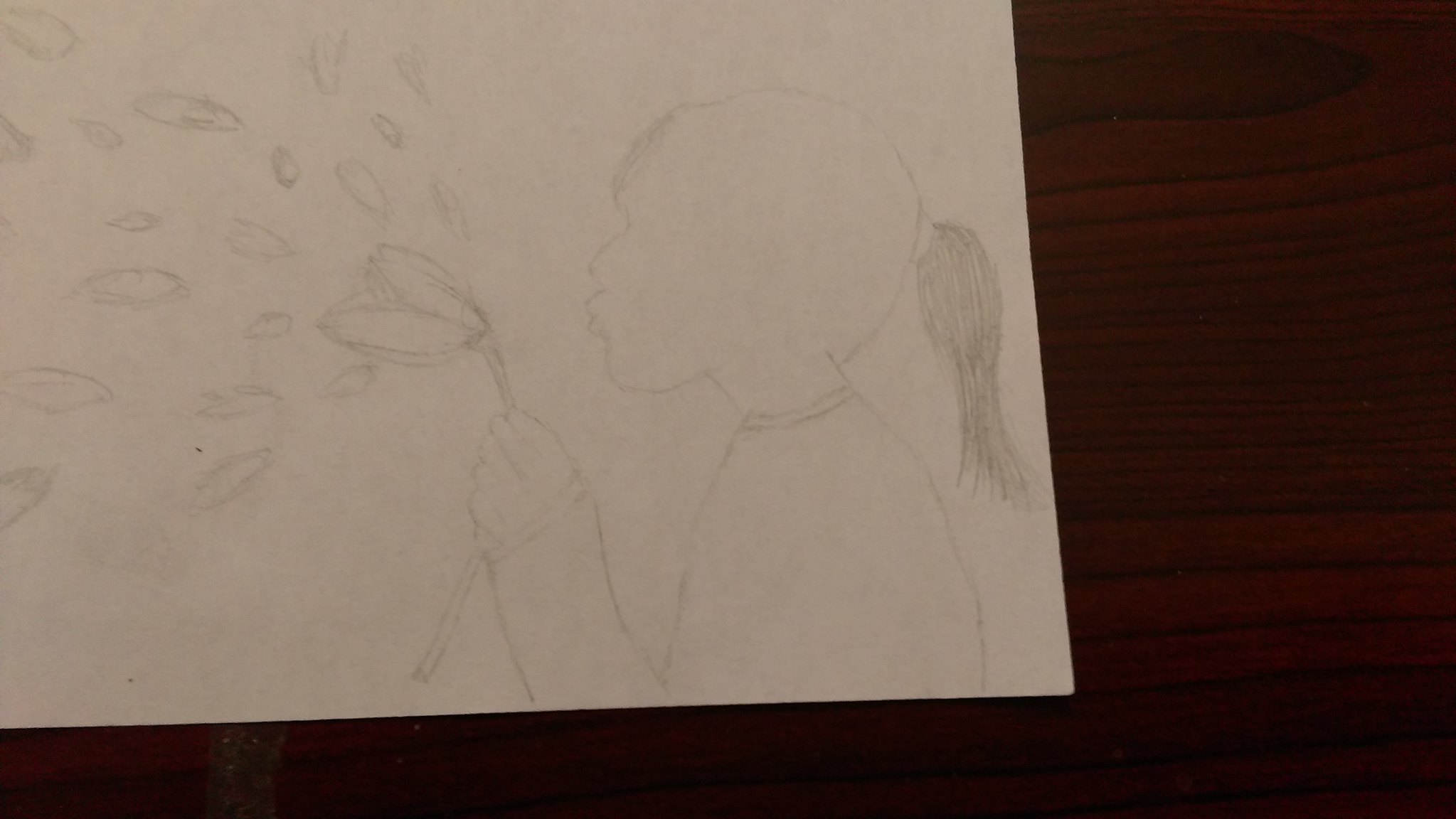The image depicts a detailed pencil sketch on a white piece of paper, which appears to be laid on a very dark wooden table with noticeable wood grains. The drawing features a side view of a young girl with a ponytail extending just past her shoulders. The girl, wearing a long-sleeved shirt, is holding a flower, likely a dandelion, in her left hand. Her hand grips a stem approximately five inches long. The girl's lips are puckered as if she is blowing, and numerous oval-shaped petals are seen scattering away from the flower into the distance. The precise details capture the motion and delicate nature of the scene, while the absence of detailed facial features emphasizes the artistic simplicity of the sketch.